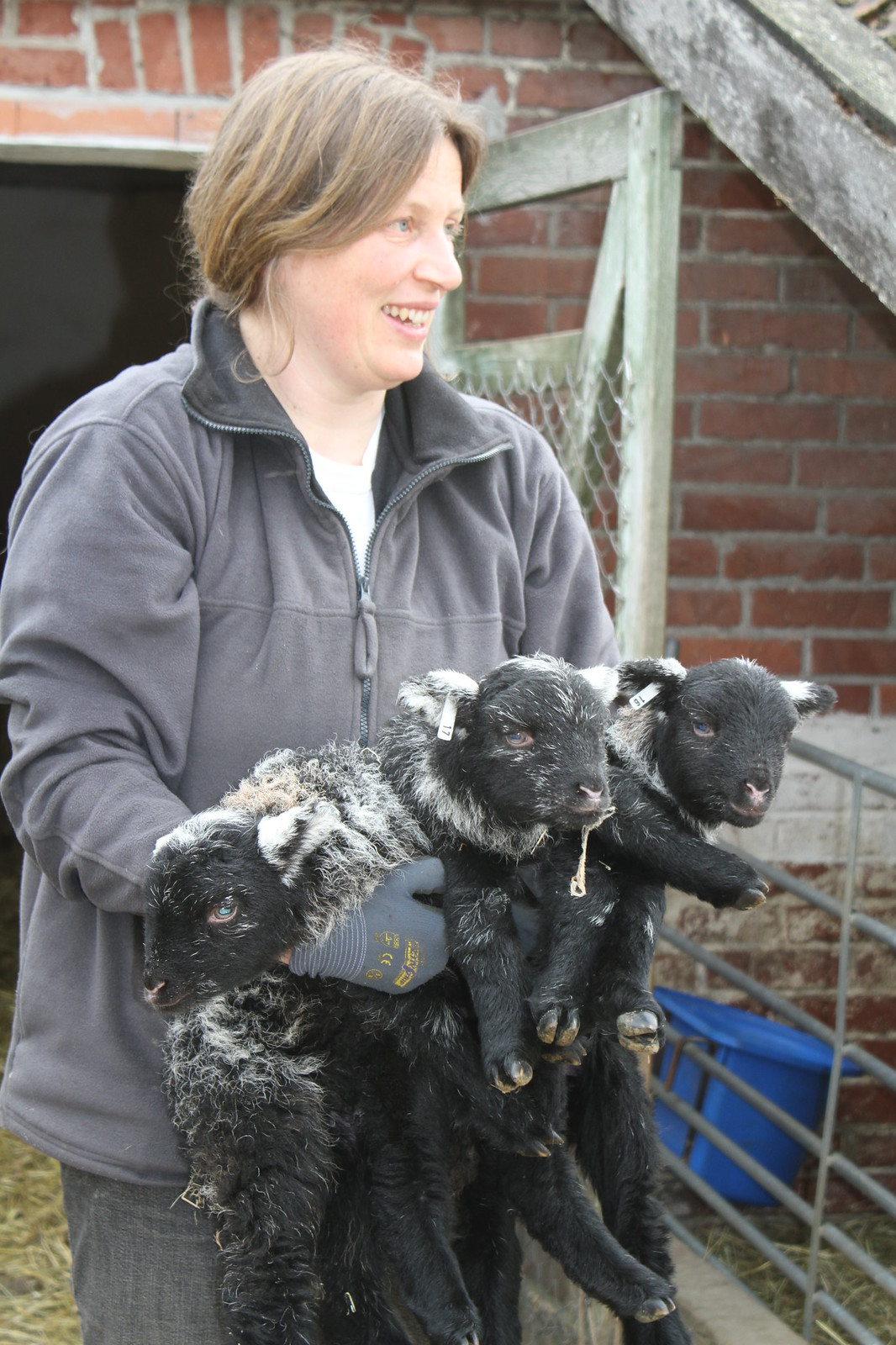In this outdoor photograph, a middle-aged Caucasian woman, smiling and looking off to the right, stands in front of a rustic, weathered wooden door attached to a brick building. She is holding three young black-faced lambs with mixed black and white fur, nestled in her arms. The woman has brown hair pulled back and is wearing a gray fleece jacket, a t-shirt underneath, gray gloves, and gray or blue jeans. One of the lambs has drool hanging from its mouth and their ears are tagged. To the right of her, a blue bucket, likely used for sheep feed, hangs on a metal fence enclosing a grazing area covered in hay.